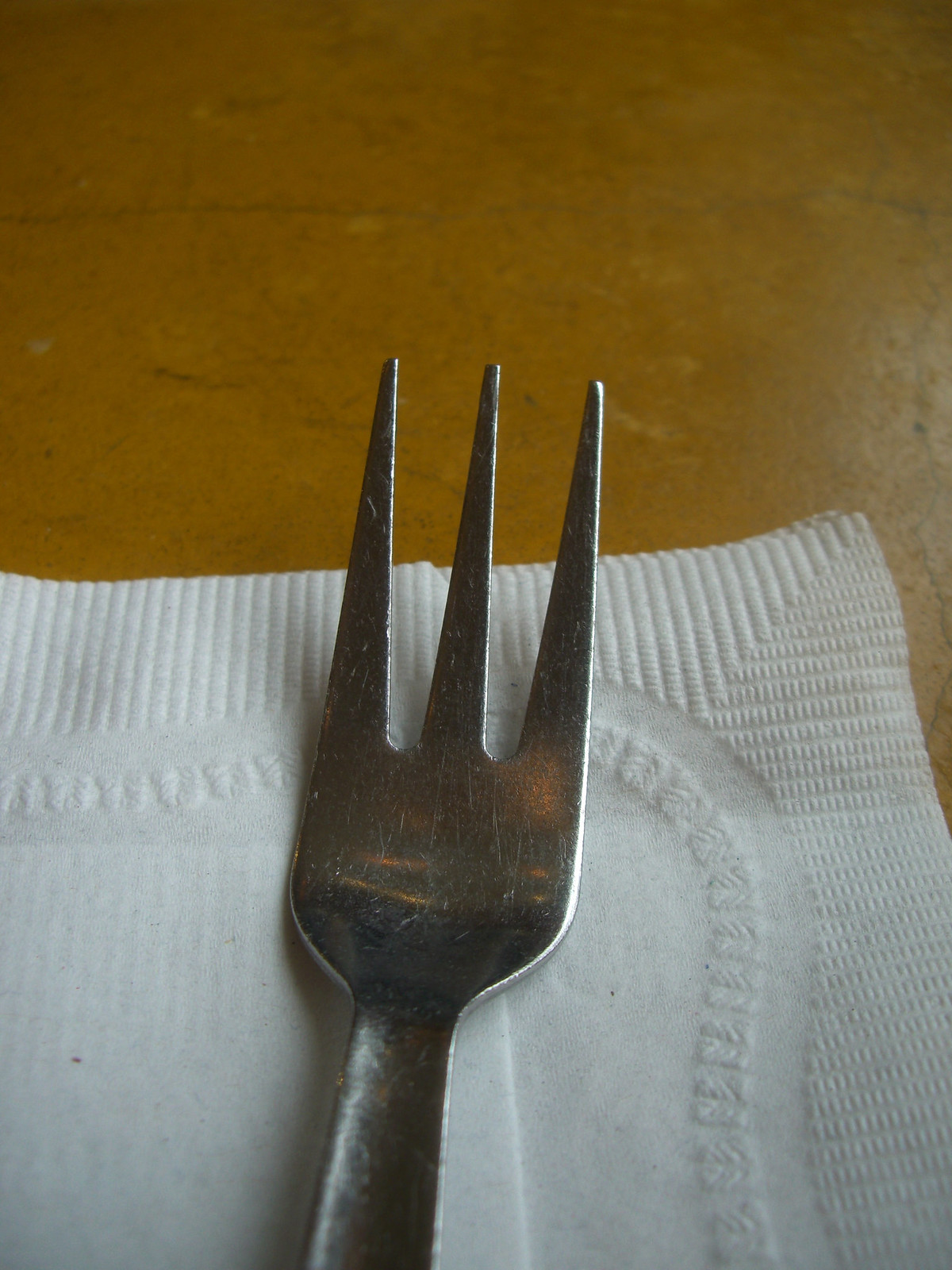This photograph captures a detailed, close-up view of a lightly aged, light brown wooden table with a few black marks, emphasizing its well-used condition. The background takes up the upper half of the image and contrasts with the bottom portion, which features a decorative white napkin laid out diagonally. The napkin is embossed with straight lines along the edges that form a neat border. At the upper edge of the napkin, near the center of the photograph, lies a simple, polished, silver fork with three tines, positioned tine-side up. The handle of the fork starts from the lower left corner of the image and extends towards the center. Faint scratches on the fork indicate it is well-used. A reflection of light is noticeable on the right-hand side of the table, adding a subtle highlight to the composition.